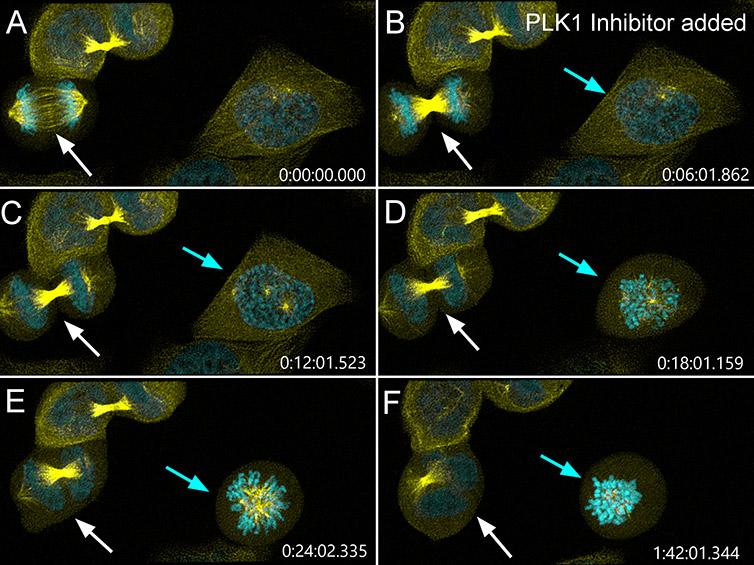The image depicts an array of six segments arranged in two rows, each labeled A through F in their top left corners. The segments portray microorganism-like cellular shapes in various colors, including bright and dark shades of blue, yellow, black, white, and gray. The cellular structures appear under a microscope-like setting with PLK1 inhibitor added, particularly noted in segment B. Each segment is distinctively coloration: goldish, teal blue, and bright blue clusters are prominent. 

The segments also have timestamps in their bottom right corners: A (0), B (601862), C (1201523), D (1801159), and E (2402335). The cellular formations transition from yellow and black shapes to bright blue with clusters showing an orange or yellow center as you move across the segments. White lines delineate each segment, and small arrows point at the cellular shapes indicating areas of interest or change within each segment.